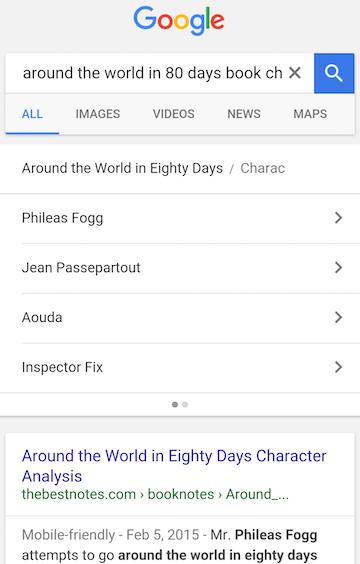The image showcases a Google search results page for the term "Around the World in 80 Days book." At the top, there is a prominent search bar paired with a blue and white search icon. Directly below, the search results feature the title "Around the World in 80 Days," followed by a list of key characters: Phileas Fogg, Jean Passepartout (listed here as Gene Passit), Aouda, and Inspector Fix. Two dots, one dark gray and one light gray, are positioned underneath this list. 

Further down the page, there's a search result linking to "thebestnotes.com" with the description "Mobile Friendly, February 5, 2015," noting that Mr. Phileas Fogg attempts to circumnavigate the globe in 80 days. The navigation tabs near the top of the search results include options for Images, Videos, News, Maps, and a highlighted "All" tab, which is blue with an underline to indicate it is currently selected.